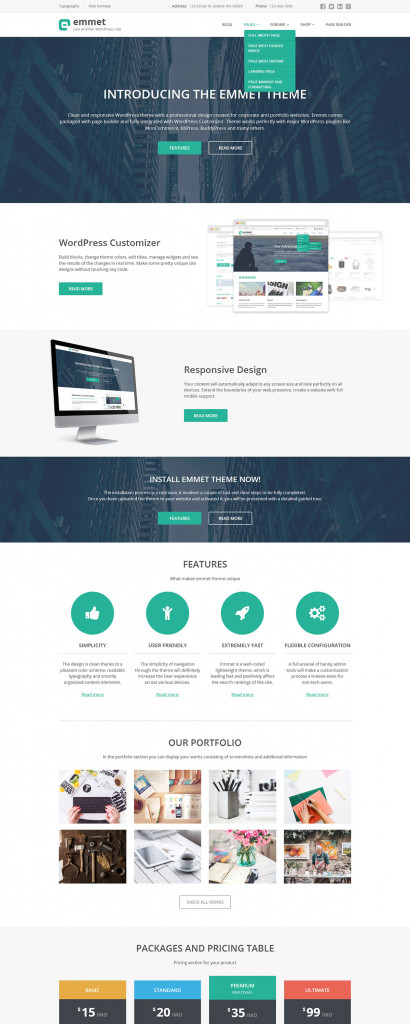**Caption:**

The website showcases the WordPress theme 'Emmet.' At the top-left corner, you'll find the Emmet logo, which features a green, almost complete circular design missing the lower right-hand corner, with a green dot at its center. Right next to the logo, the name "Emmet" is prominently displayed. To the right of this, there is a navigation menu with several drop-down options.

The header section of the site displays an urban skyline background with the text "Introducing the Emmet Theme," accompanied by some descriptive text and buttons for exploring features or reading more. Following this is a section explaining that Emmet integrates seamlessly with the WordPress customizer, offering additional text, a call-to-action button, and an image showcasing various theme layouts.

Further down, the site elaborates on the theme's responsive design with detailed descriptions and another button for further information. Additional sections guide users on how to install the theme and delve into its various features.

Towards the bottom, the website presents a portfolio featuring images of different theme layouts followed by a packages and pricing table.